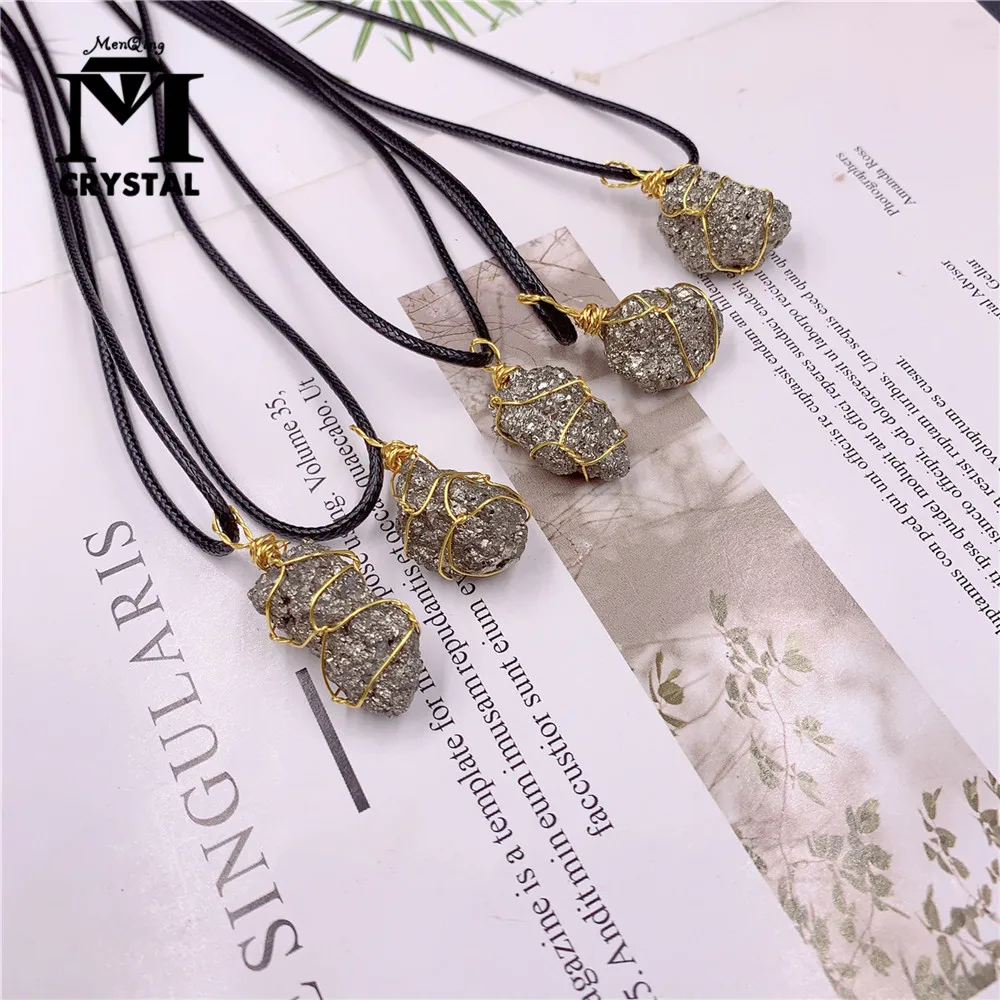This detailed photograph showcases five necklaces elegantly arranged on an open book adorned with artistic black text and illustrations of leaves and branches. Each necklace is composed of a black nylon cord and features a pendant made from natural, irregularly shaped stones. These stones exhibit a silvery, shiny, and glittery surface, akin to dark gray granite with a noticeable sheen. The stones are each encased in a thin golden wire that wraps around them multiple times, forming intricate coils and intertwines. The wire also curls around itself to create a hoop, connecting the pendant to the cord. Notably, the book underneath prominently displays a large 'M' and the word 'crystal,' possibly suggesting that these stones are some type of natural crystal. The entire setup is artistically pleasing, with the reflective stones and their golden wire settings offering a visual contrast against the black cords and the creatively illustrated background.